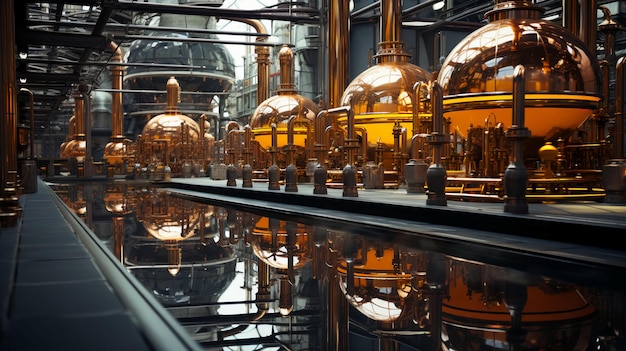The image depicts a sophisticated, potentially computer-generated, steampunk-like factory interior, reminiscent of a scene from "Willy Wonka and the Chocolate Factory." Dominating the background are at least six enormous, shiny brass spherical containers, some reports suggest up to seven, with large pipes interconnecting them and extending out of the frame. These containers, likely kettles or chemistry beakers, exude an intricate, detailed design with their semi-transparent or reflective surfaces. Shadows from these kettles cast striking reflections in a narrow, highly reflective body of liquid, possibly water or an alcohol still. This liquid pool runs diagonally from the bottom right of the image to the left. The entire scene features a complex array of equipment and sleek brass pipes, with part of the structure seemingly set outdoors. The factory exudes a new, polished look, devoid of any human presence, with a detailed and meticulously crafted ambiance. Rafters are visible, supporting the indication of an industrial setting. Additionally, non-brass gray tanks and structures contribute to a dual-colored theme of amber and gray, enhancing the overall sophisticated aesthetic of the factory.